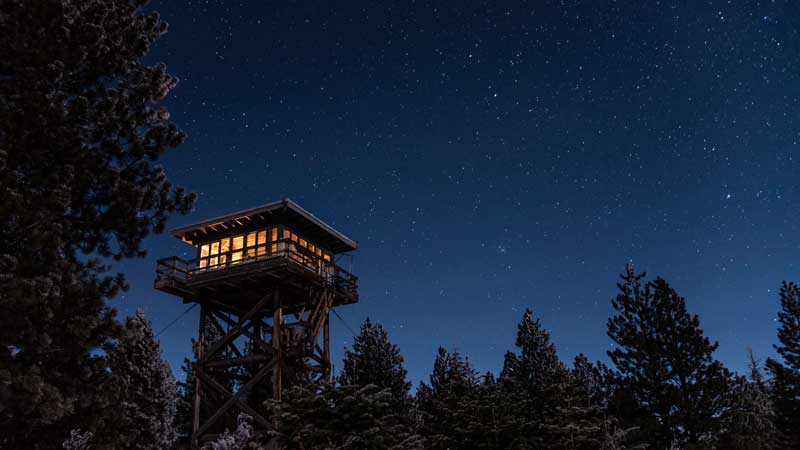The photograph captures a serene, picturesque night scene in a dense forest of towering evergreen and pine trees, resembling giant Christmas trees. Positioned slightly to the left of center, a large and cozy fire tower or ranger post stands majestically. Constructed from wood, it features a zigzagging staircase leading to the top, where a spacious, cabin-style structure awaits. This top section is warmly lit from within, casting an inviting orange-yellow glow through the numerous windows — a sign of possible occupancy. The structure also boasts a wraparound porch and an overhanging roof, enhancing its allure as a potential vacation spot rather than just a functional observation post. Overhead, the sky is a blanket of stars, dazzling in its clarity and adding to the tranquil beauty of the scene. The overall composition is one of serene wilderness juxtaposed with the cozy, illuminated lookout, offering a perfect blend of natural splendor and human comfort.